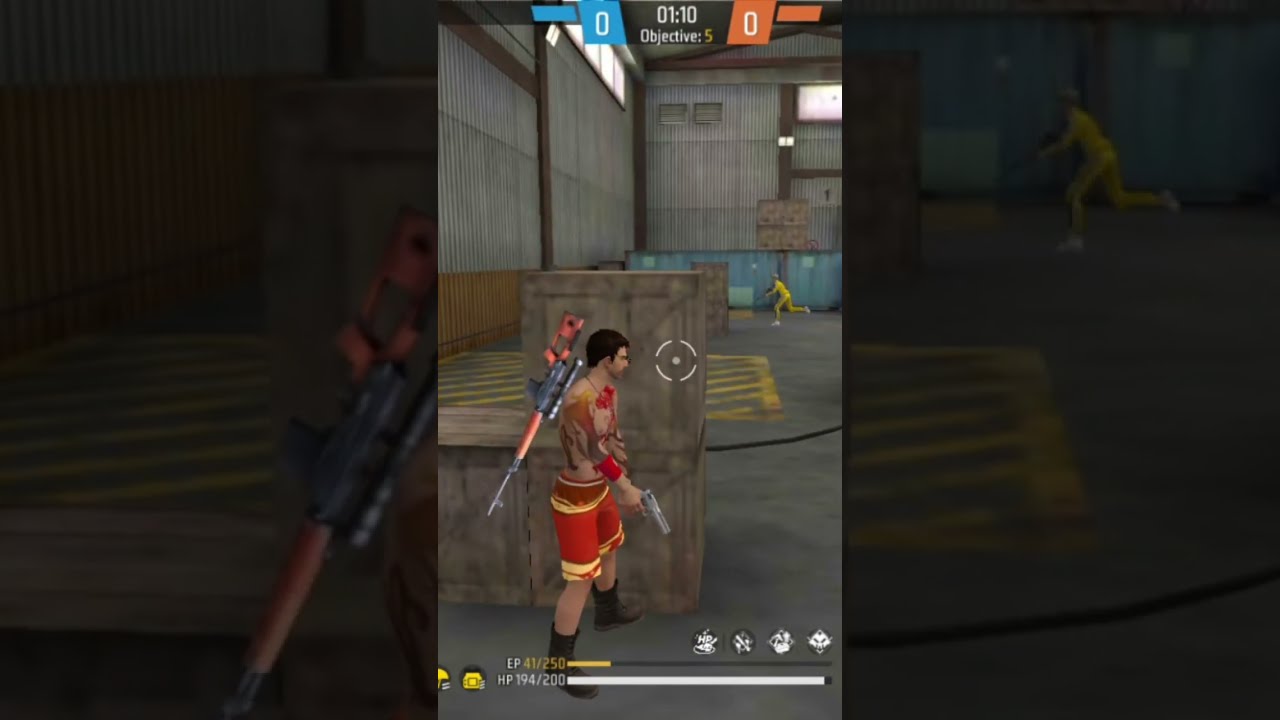The image is a horizontally rectangular, three-panel shot from a video game set inside a warehouse. The scene is full color, with the small, bright center panel flanked by larger, darker zoom-ins of the same image. The warehouse features corrugated metal walls, supported by dark brown beams, with light streaming in through high windows. The concrete floor has yellow-striped painted areas and there are various brown crates scattered around. The focus is a man with yellow and red tattoos, wearing matching shorts and black boots. He wields a handgun in his right hand and carries a red and gray rifle on his back. Positioned behind three large gray crates, he appears to be hiding from a competitor dressed in a yellow suit seen running in the background. Additionally, the top of the image displays a timer at 1 minute and 10 seconds, with an objective marker showing "Objective 5" and a score of 0 for blue and 0 for orange.